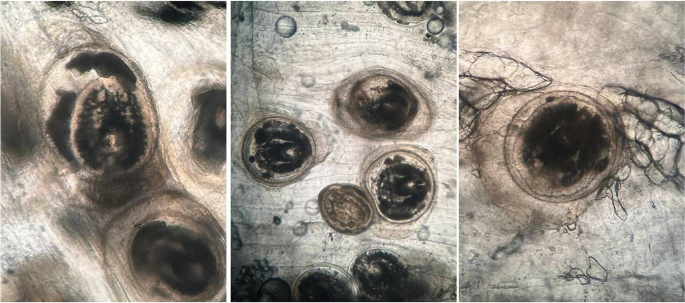The image consists of three microscopic pictures arranged side by side in a row. Each picture depicts cells or microorganisms with a recurring color palette of black, brown, and gray. 

In the leftmost picture, two round cells are prominently featured. These cells are primarily black and brown, surrounded by a mix of white, brown, and black areas. 

The central picture showcases four cells in total, with three prominent cells in the middle and additional cells on the sides. The three central cells are mostly black, while the fourth central cell is smaller and brown. The background is a blend of white and gray with noticeable bubbles interspersed.

The rightmost picture shows a single round cell, mainly black and brown, in close-up detail. Surrounding this cell are vacuole-like structures, and the image includes a background teeming with lighter colored bubbles. Additionally, there seems to be veiny black material present.

All three images depict a microscopic environment with cells immersed in a liquid medium, characterized by the recurring appearance of circular bubbles and intricate cellular structures.